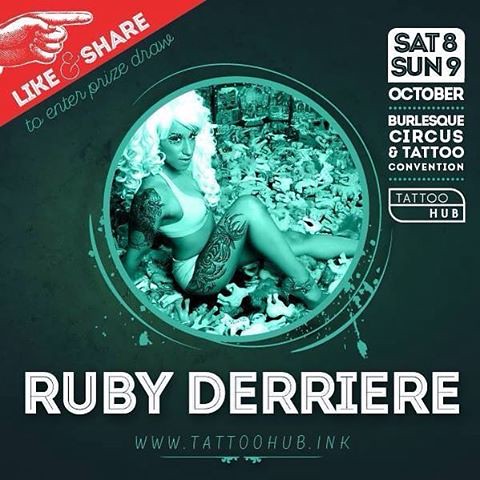In the center of the square image, set against a dark teal background, an attractive woman in a white bikini top and bottoms strikes a pin-up pose. Her platinum blonde wig complements her high-heeled shoes. Her upper arms and thighs are elaborately tattooed. The woman is sitting on the ground, framed within a tinted teal circle, and surrounded by what appear to be tiny horse toys, possibly My Little Ponies. A promotional event, "October Burlesque Circus and Tattoo Convention," spans the upper right corner, with "Saturday 8th, Sunday 9th" also noted. In the upper left, a red section features a hand pointing right and the phrase "Like and Share." Below the woman's image, bold text reads "Ruby Derriere" along with the website "www.tattoohub.inc."